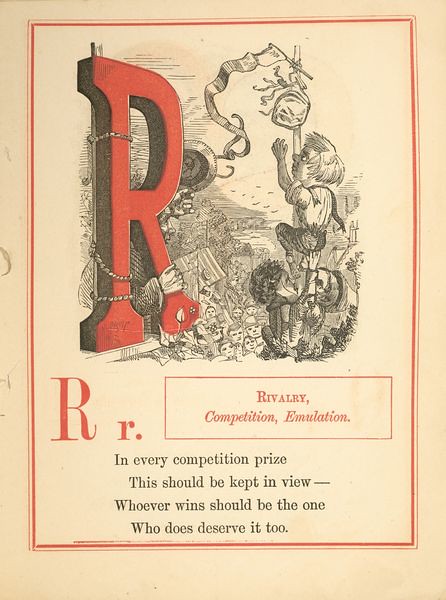This rectangular image, likely from an old book or magazine, measures approximately 4-5 inches tall and 3-4 inches wide. The page has yellowed with age and is framed by two red pinstripe outlines. The top half features a black-and-white illustration with a prominent large red letter "R" on the left side, appearing three-dimensional. This "R" is being held by a man who is waving a hat towards several boys on the right, who are energetically climbing a pole. At the top of the pole, there appears to be a flag or bag that the boys are reaching for. Below this illustration, there's a red capital "R" followed by a lowercase "r" with a period next to it on the left. Next to this is a small, wider-than-tall rectangle with a red border that contains the words "Rivalry, Competition, Emulation" in red text. Further down, in small black print spread over four lines, it reads: "In every competition prize, this should be kept in view. Whoever wins should be the one who does deserve it, too." The image's red motif and competitive theme suggest branding related to a sports team or event, possibly the Rovers team.